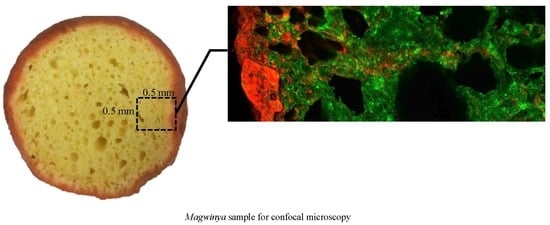The image showcases two distinct sections. On the left side, there is a circular object resembling a piece of garlic bread or a flat crouton, with a browning outer crust and a buttery yellow interior dotted with small pockets. This object displays craters and herb flakes, contributing to its irregular yet rounded shape. A small black square labeled "0.5 mm" on both the top and left sides is imposed on the object, indicating a dimension reference. A line extends from this square towards the top right, leading to a zoomed-in rectangular image on the right side of the overall picture.

The right section features a close-up view of the highlighted area from the left object. This magnified image reveals intricate green strands with orange edges where the crust appears, set against a black background. The detailed texture suggests a microscopic examination of the surface. Below this zoomed-in depiction, the text reads "MAG WINRAR SAMPLE FOR CONFOCAL MICROSCOPY," indicating the technical nature of the image analysis.